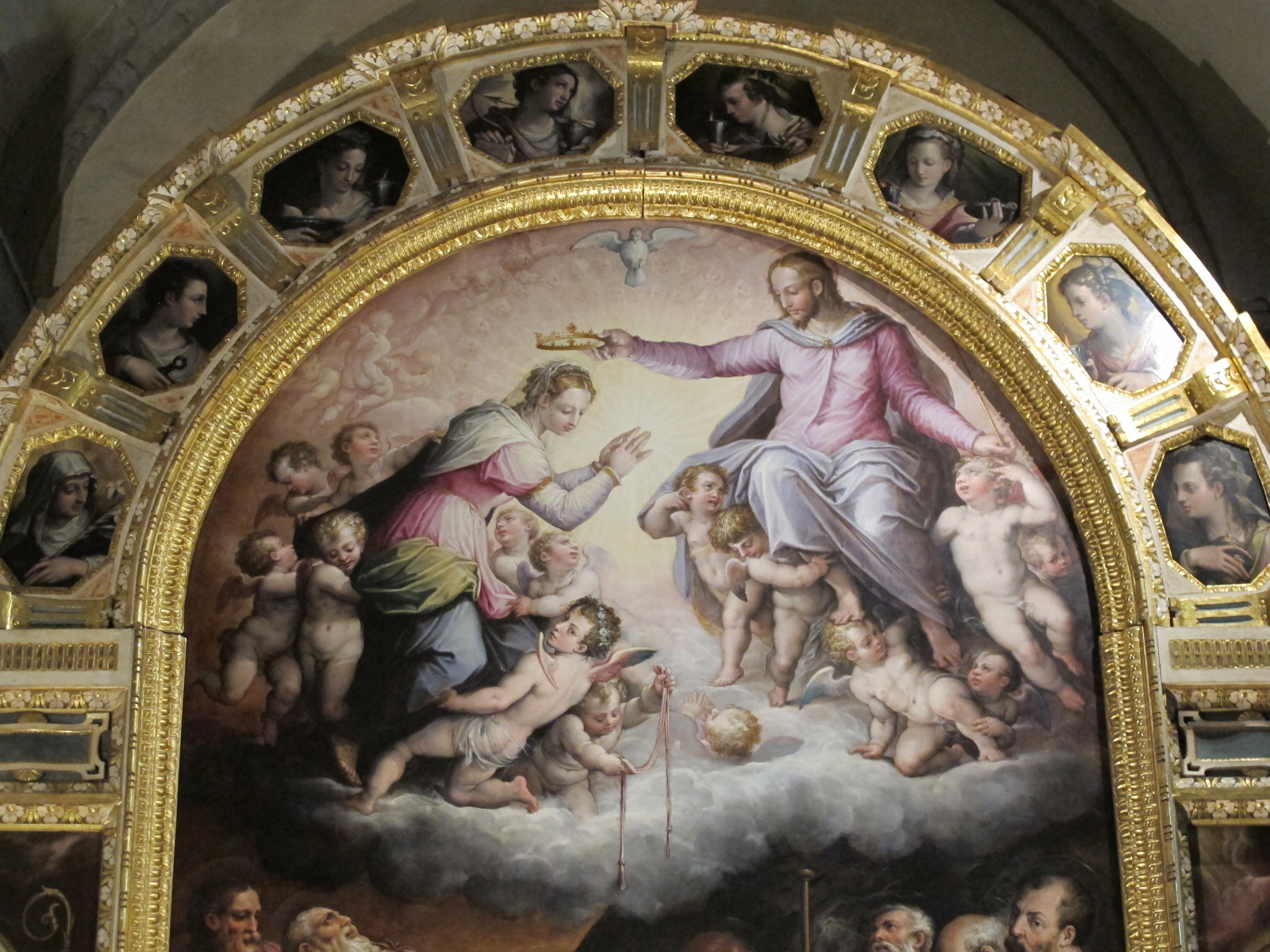The image depicts an intricate religious painting set within the arch of a church. The arch itself is adorned with a golden and ivory border featuring floral designs and a rope-like texture. Along the border are smaller portraits of various men and women dressed in formal garb, seven to eight in total. The central painting showcases a man, often interpreted as Jesus, seated on a cloud and surrounded by numerous cherubic angels. Dressed in a purplish-pinkish and bluish robe, he is crowning a woman to his left, also robed similarly. The woman, possibly in an act of reverence or acceptance, raises her hands and gazes downward, seemingly distracted by the little cherubs around her. Both the man and the woman are supported by the cloud of cherubs. Below them, human figures—some with beards and mustaches—look upwards from beneath the cloud. Crowning the entire scene at the top of the arch is a white dove, symbolizing the Holy Ghost, against a light brown sky. The painting intricately combines elements of divinity, reverence, and celestial beings within a richly detailed and ornate arch.